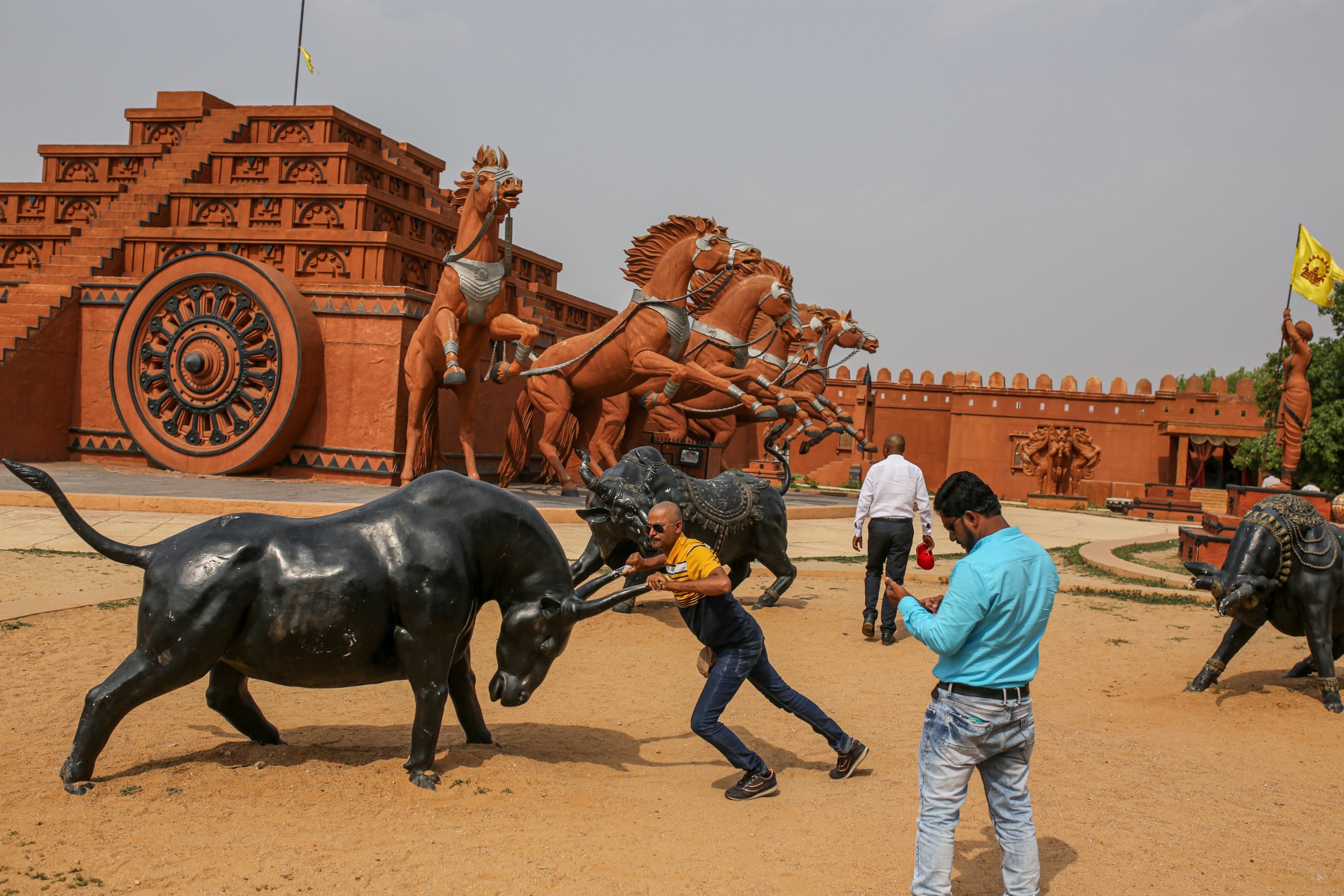In this rectangular photograph, a man poses for a picture, grabbing the horns of a black bronze bull statue situated in a sandy pit. He wears dark blue denim pants and a short-sleeved black and yellow shirt, appearing as if engaged in a playful wrestling match with the bull. To his right stands another man, dressed in blue jeans and a long-sleeved blue shirt, looking down at his phone, possibly preparing to capture the moment. 

In the background, a man in black dress pants and a long-sleeved white shirt can be seen walking away from the scene. Behind them, a small South American-style pyramid with five rungs ascends from ground level, featuring a central staircase and a large castle-like structure adorned with rearing, majestic dark brown horse statues. Atop the pyramid, a statue of a man holding a yellow flag with a brown circle is visible. The photograph highlights a collection of statues within a sandy and dirt-filled area, bordered by sidewalks and framed against a backdrop of a large brown wall with white dots and spikes at the top.